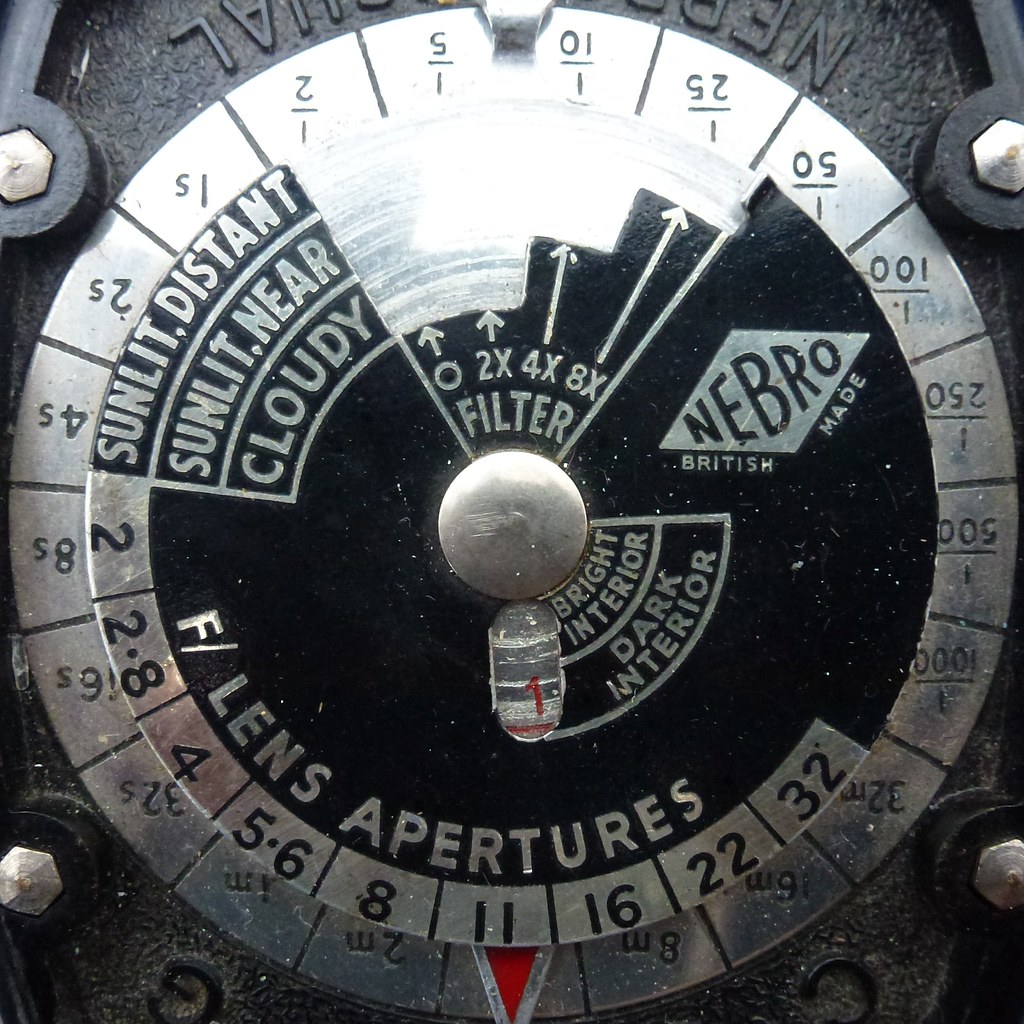The image displays a detailed Nebro British-made film lens aperture, centrally positioned within a gray and black metal fixture. The metal dial is round, with a black interior and various inscriptions highlighting its functions and settings. Notably, the black circular portion of the aperture is labeled with "sunlit distant," "sunlit near," and "cloudy." Adjacent to these markings are filter settings denoted by "0," "2x," "4x," and "8x," each with corresponding arrows. Additionally, a white diamond shape prominently displays the brand "Nebro, British made."

Surrounding the dial are multiple series of numbers printed along the metal edge, indicating measurement values in millimeters. Labels for "bright interior" and "dark interior" are also present, providing crucial information for photographers aiming to achieve optimal lighting conditions. The entire assembly is secured by four bolts at the corners of the image, integrating the lens aperture firmly into the metal background. The overall color scheme predominantly features shades of gray, black, and hints of red, creating a stark, industrial aesthetic.